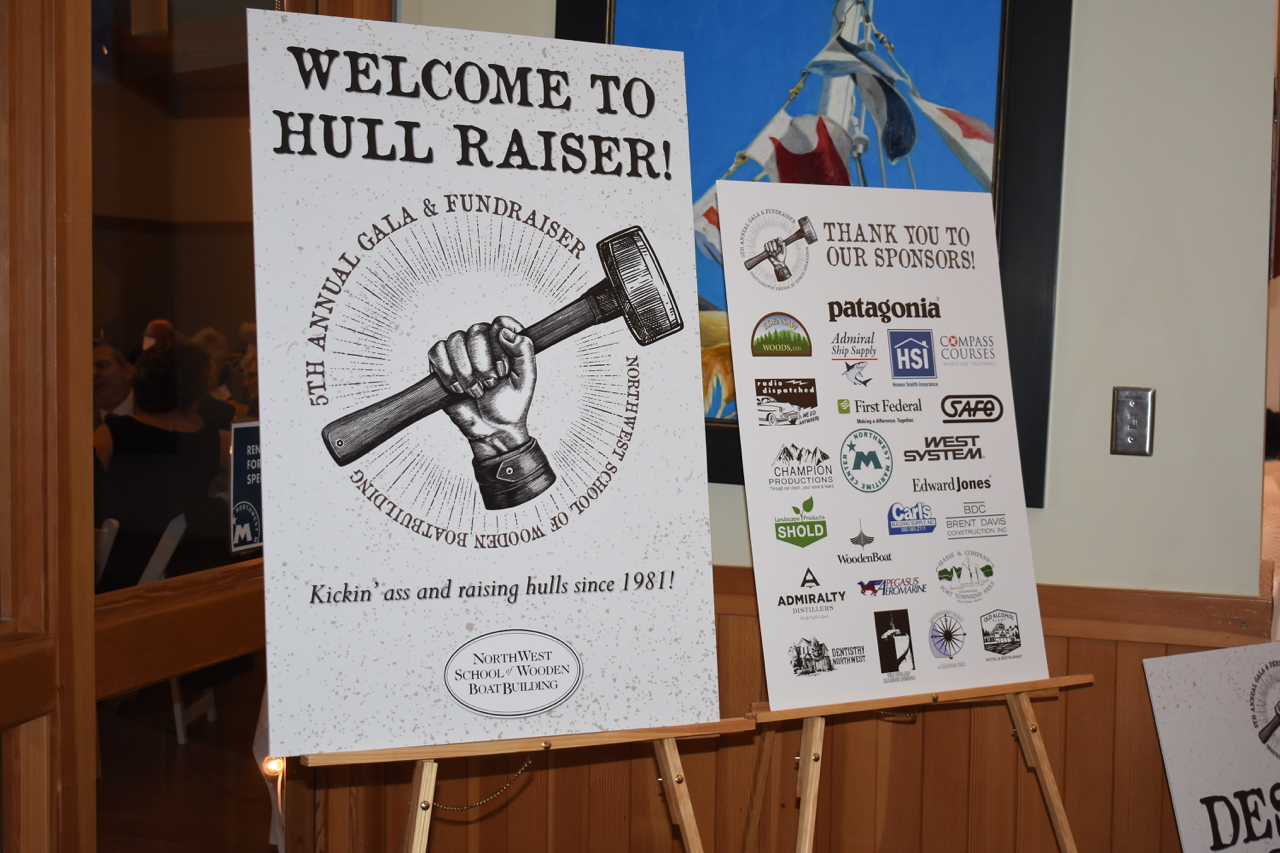The image showcases two wooden easels positioned in a setting that appears to be a library or museum room, accentuated by wood paneling and glass elements in the background. The first easel displays a striking sign featuring a hand gripping a sledgehammer, set against a white backdrop, with black text proclaiming, "Welcome to Hull Razor, kicking ass and raising hulls since 1981." This sign also references the fifth annual gala and fundraiser for the Northwest School of Wooden Boat Building, accentuating their theme, "Northwest Strong." Adjacent, the second easel supports a sign laden with an array of sponsor logos, headlined with a "Thank you to our sponsors." Notable names such as Patagonia, Schold, and Carl's West System are visible, emphasizing the event's community support. The setting is further detailed with finer touches like an electrical outlet and partial signage reading "DES," adding to the authentic and detailed atmosphere of the scene.